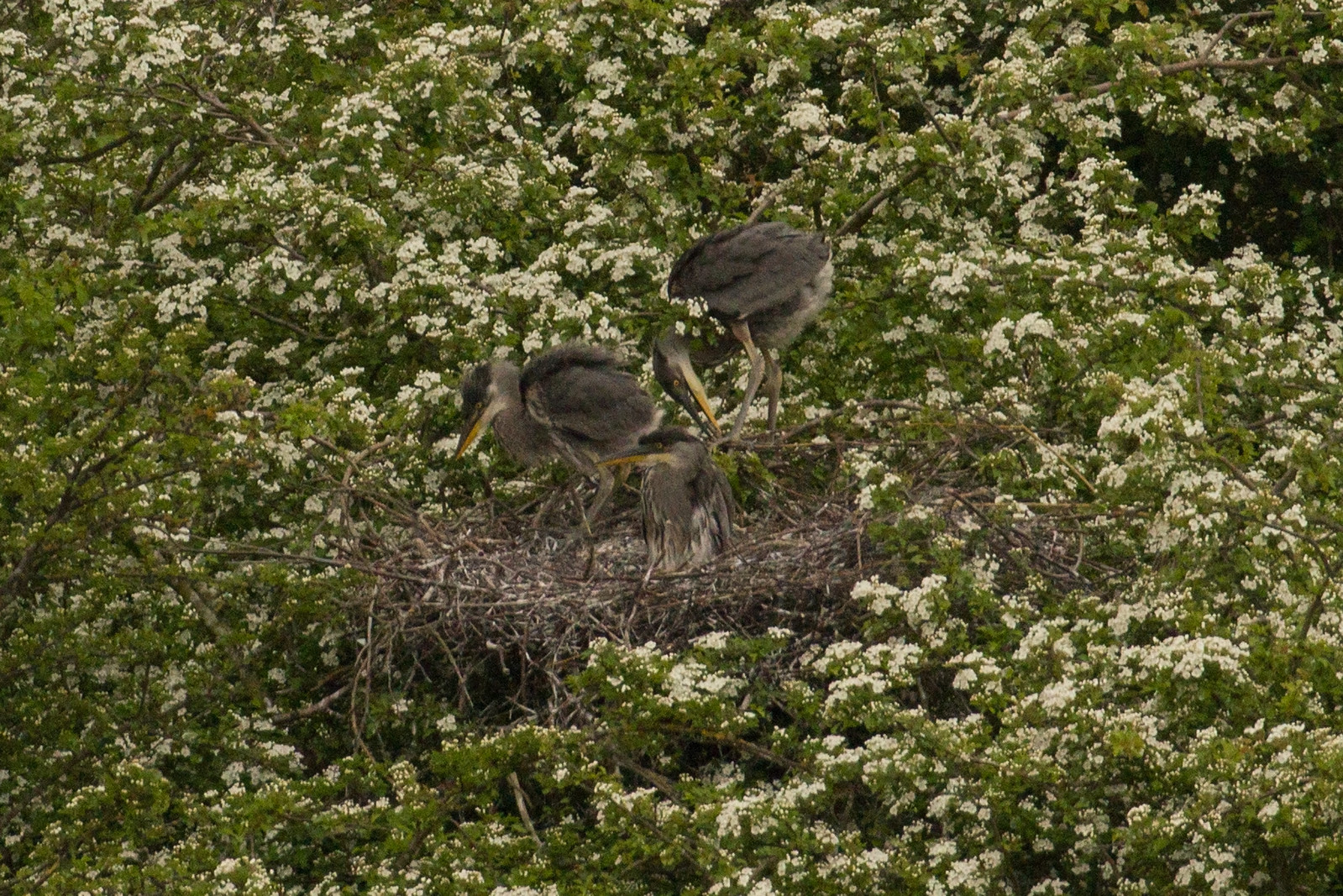A close-up photograph of a lush tree whose leafy canopy fills the entire background. The tree is adorned with clusters of tiny white flowers and possibly some small white berries interwoven among its vibrant green leaves. Nestled in the center of the image is a bird's nest composed of various thin, dark and light gray twigs. In the nest stand three birds that resemble storks. These birds have fluffy gray plumage that almost looks like fur. Their legs are light gray, and their remarkably long and pointy beaks are yellow underneath with gray tops. The bird on the far left is standing and facing left, providing a clear side view of its body. The bird in the middle is sitting, offering a frontal view of its body and a side perspective of its head. The bird on the right, which appears to be an adult, is standing and scratching its foot with its beak. Lower in the nest is a fairly large baby bird, blending into the scene with its similarly fluffy gray feathers and a distinctive black and yellow beak.